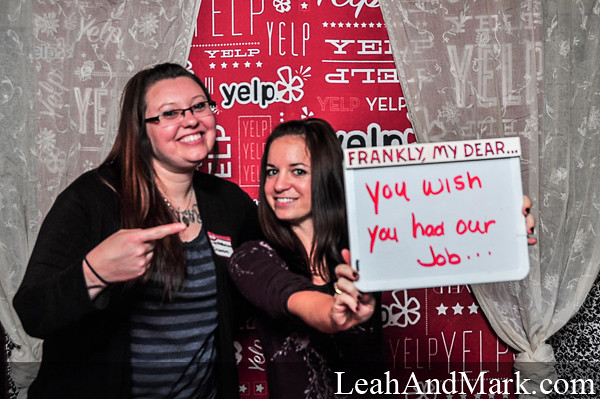The image features two young women standing in front of a backdrop decorated with multiple Yelp logos. The woman on the right has long black hair and is holding a whiteboard that reads, "Frankly, my dear, you wish you had our job," written in red marker. She is shorter than the other woman with long brown hair, who is smiling and pointing at the sign. Both women are smiling, exuding confidence. The taller woman wears a blue and gray striped shirt, while the backdrop is further adorned with white lace curtains tied at the bottom, partially obscuring the Yelp logos. At the bottom right of the image, the URL "leahandmark.com" is prominently displayed.